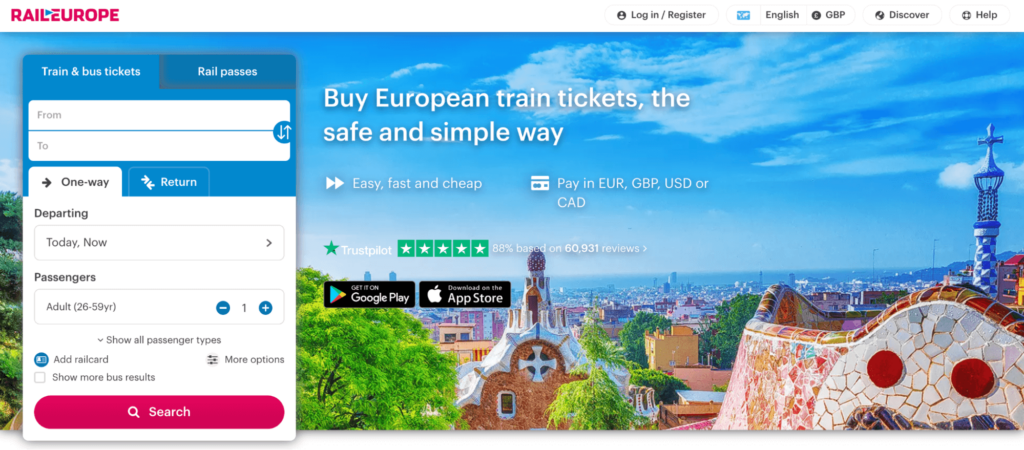A detailed caption for the described image could be:

"A panoramic screenshot of the Rail Europe website dominates the visual space, with a width approximately two and a half times its height. In the upper left corner, a prominent pink logo labeled 'RAIL EUROPE' in capital letters grabs attention. Moving rightward across the top, there are options for 'Login/Register' and a language selector currently set to 'English'. Adjacent to this, a currency dropdown indicates 'GBP', followed by navigation buttons labeled 'Discover' and 'Help'. Below this header, the main content area features an expansive banner image, overlaid with a booking form on the left. The scenic banner showcases an elevated view capturing a picturesque urban landscape. The right half of the image reveals an array of white and brown buildings dotting the skyline, alongside a distinct blue and white tower crowned with a blue cross. The horizon recedes into a gentle fog, blending the infinity of rooftops with the soft blue sky. Sparse clouds linger in the upper right corner, while verdant tree canopies peek into view from the lower left. The booking form overlay on the left suggests options for planning trips, including fields for destinations and travel preferences such as one-way or round-trip selections."